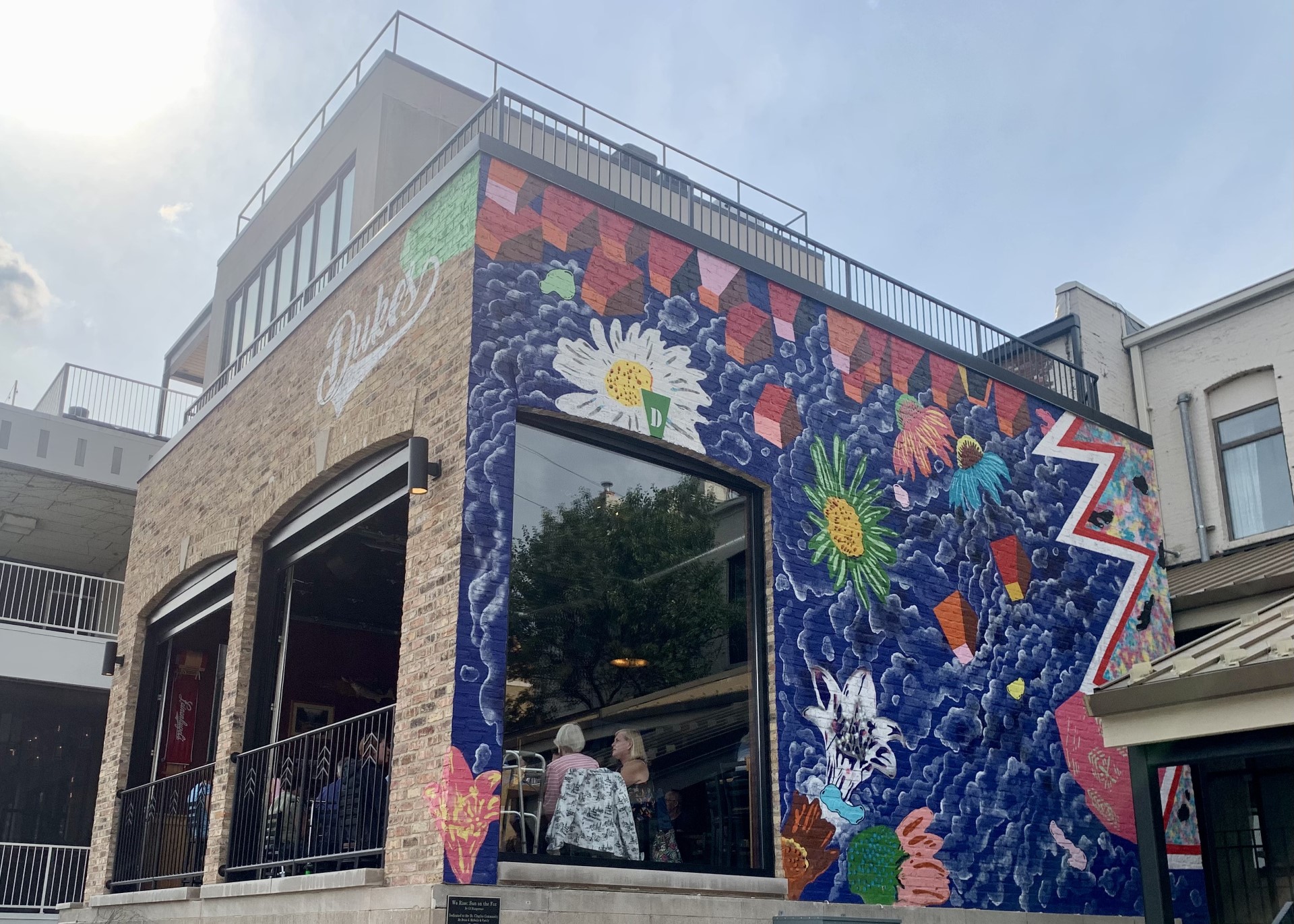This outdoor photograph captures a brightly lit street corner featuring a one-story brick building adorned with a colorful mural and a balcony on top. The building, identified as Dukes by the white script logo prominently displayed on the upper portion of the front wall, appears to be a restaurant or cafe. The mural on the viewer's right side of the building is vibrant, featuring an array of blue, orange, and green flowers, lending a tropical and spring-like atmosphere. 

The front of the building, revealed to the left in the three-quarter view, includes two open window openings offering a glimpse into the bustling interior, where several patrons are visible. A large glass window on the mural-covered side reflects parts of the exterior while revealing diners inside. Two women are seen prominently in the foreground, seated and eating near the window, while other diners can be observed further back inside the establishment. The photograph, taken on a bright sunny day with the sun positioned in the top left corner, captures the sunlit building surface in vivid detail, emphasizing the lively and inviting ambiance of Dukes.